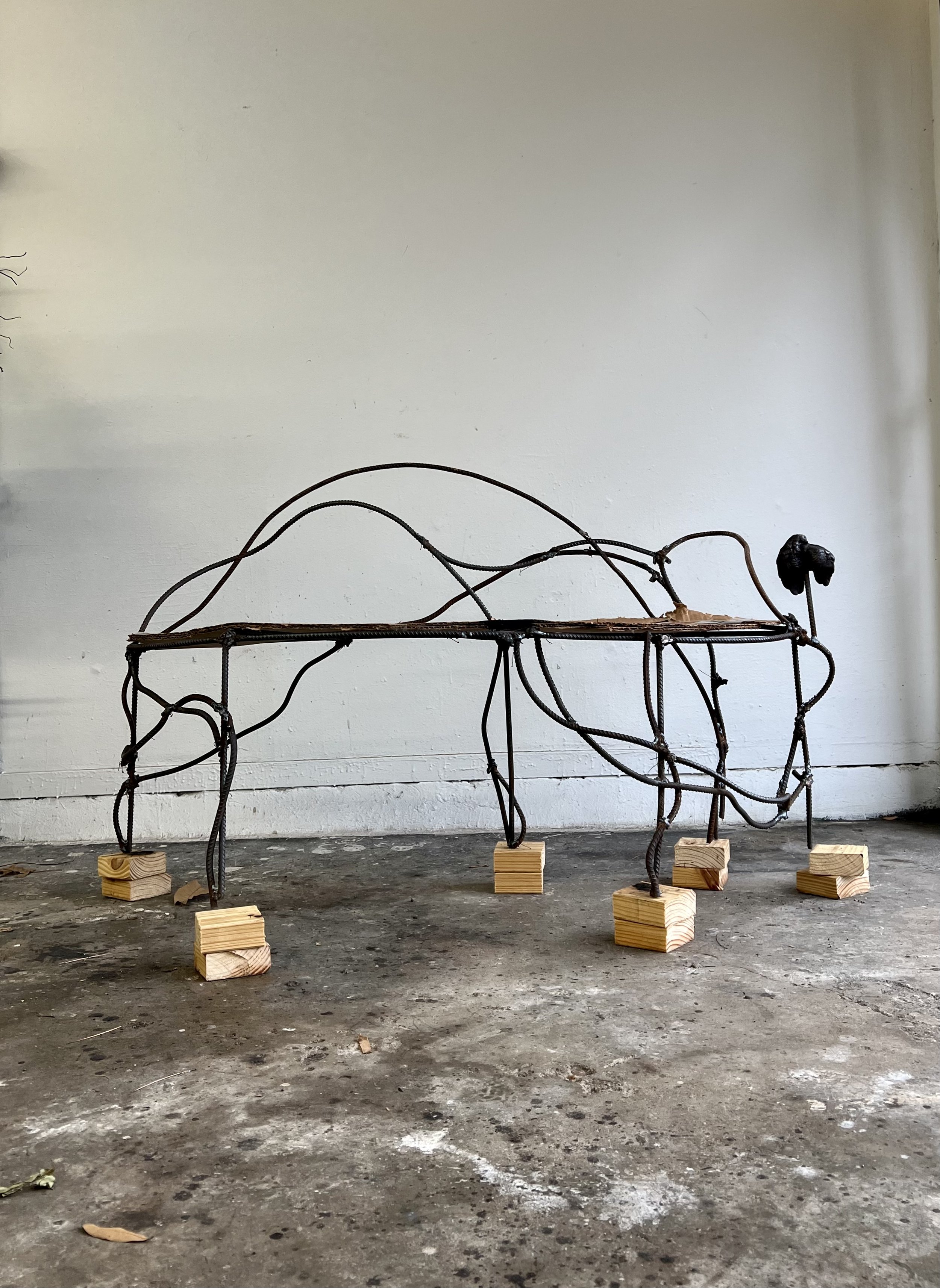This indoor photograph captures an intriguing art installation, prominently featuring a unique metallic structure that resembles an abstract animal or a distorted table. The sculpture, composed of thin, bendy metal rods, has six intricately curved legs that give it an organic yet mechanical appearance. Each leg is delicately placed on small, square, paired wooden blocks, adding to the structure’s surreal and artistic ambiance. The setting of the image reinforces the artistic vibe, as the gray cement floor beneath the sculpture is speckled with white paint or dust, creating a somewhat dirty and rustic studio atmosphere. The background is a plain white wall, which contrasts with the complexity of the metal structure, further highlighting its intricate design. Each metal rod seems to extend and swirl around a flat base area, contributing to the artistic and unfinished feel of the installation. The overall scene appears to be a work in progress, evoking curiosity and admiration for the creativity behind the piece.